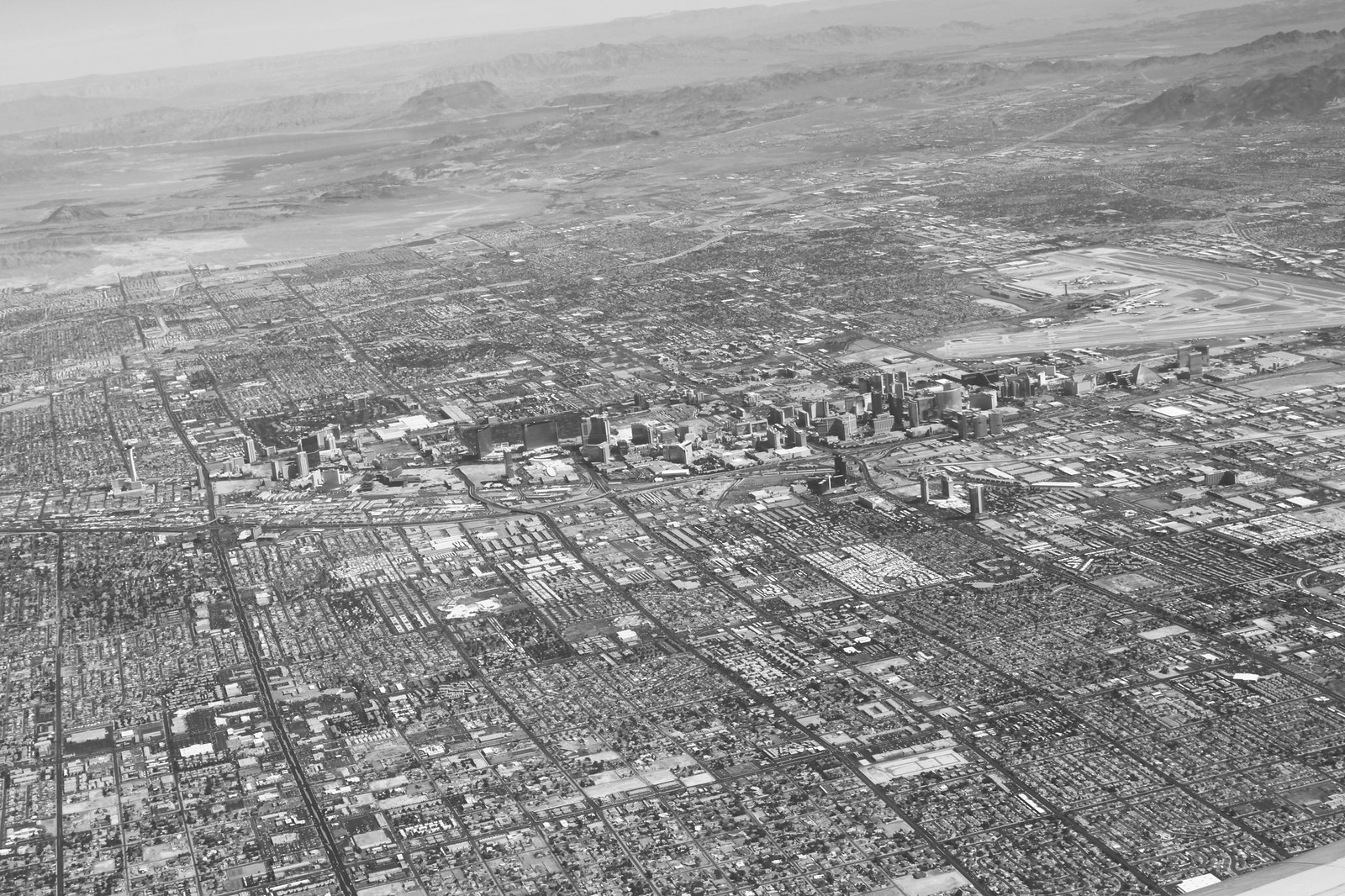The black and white aerial photograph captures a city nestled within a semi-arid or desert region, characterized by its dry, rugged mountains encircling the urban sprawl. Dominating the center of the image is a compact downtown area with tall buildings prominently clustered together. Surrounding this dense core, a grid network of possible residential areas extends outward, punctuated by intersecting main thoroughfares. Sparse vegetation, with few trees in sight, accentuates the arid nature of the landscape.

A layer of dust or haze, perhaps stemming from pollution, hangs over the scene, casting a muted, almost vintage atmosphere. The city seems relatively underdeveloped, with minimal modern infrastructure, suggesting it could be an outlying area or captured in a bygone era. The surrounding terrain hints at large salt lakes and potential mining activities, further emphasizing the industrial undertones of this enigmatic locale.